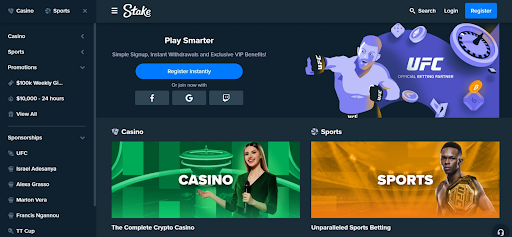A detailed snapshot of the Stake app interface is depicted. At the top, the app name "Stake" is prominently displayed. Below are various interactive buttons for categories such as UFC, represented with an illustration of a boxer wearing punching gloves. Accompanying the fighter's image is a roulette wheel, dice, and poker chips, hinting at gaming options. 

Further down, there's a section for the Casino, featuring a lady against a green background, pointing towards a roulette wheel. This area is adorned with various decorative arches. Adjacent to the Casino section is the Sports area, where another boxer is illustrated with a determined expression. The boxer is set against an orange background with lights that suggest an arena setting.

The slogan "Play Smarter" is prominently placed above a blue button labeled "Register," whose subsequent text is not clearly visible. On the left side of the interface, there's a toolbar with quick access icons for the Casino, Sports, and Promotions, among others. The headings in smaller text such as "Sponsorships" and "UFC" are difficult to read clearly.